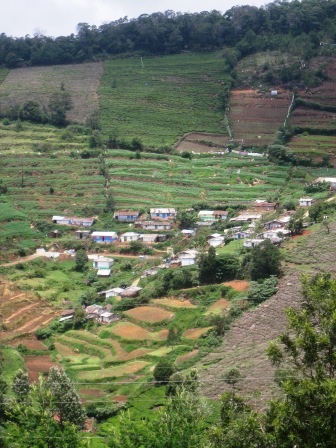The image depicts an overhead, albeit sideways-tilted, view of a small village nestled within a lush valley. The tilt disorients the viewer, positioning the sky to the right and tree-covered terrain to the left. Dominating the scene, terraces rise steeply from the valley floor, resembling vast, agricultural steps, reminiscent of South American coffee fields. These terraces suggest intensive, tiered farming practices that stretch across the hillside, transforming the landscape into a series of cultivated levels. At the heart of this verdant arrangement lies a tight cluster of houses and small structures, signifying a bustling rural community enveloped by varying shades of green. The fields are variably sectioned—some into large pastures, others medium-sized, and some into precise rows—highlighting diverse agricultural activities. A dense line of dark green trees borders the horizon beneath the sideways sky, contrasting sharply with the medium-green pastures and crops closer to the camera, completing the picturesque rural valley scene.